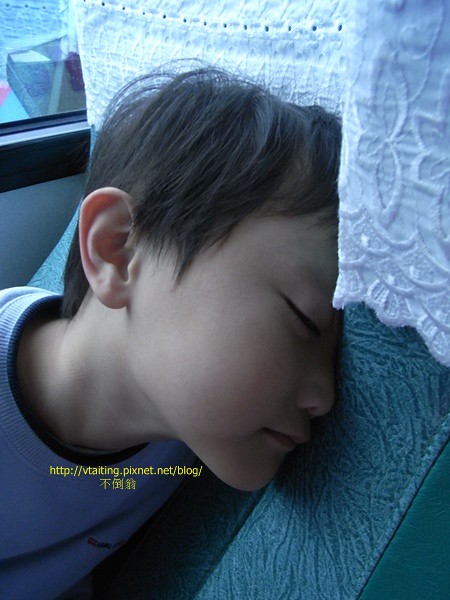This photo captures an Asian child sleeping in what appears to be an upholstered seat, possibly in a charter bus or similar transportation vehicle. The seat is green with paisley designs and has a slightly plasticky texture, complemented by a white cloth overlay on the headrest area. The child, dressed in a gray sweatshirt with a navy-trimmed collar, is peacefully propped up against the seat. Behind him, a window is visible, although it's unclear what kind of window it is. The image contains a link at the bottom, "vtaiting.pixnet.net/blog," accompanied by Asian characters.